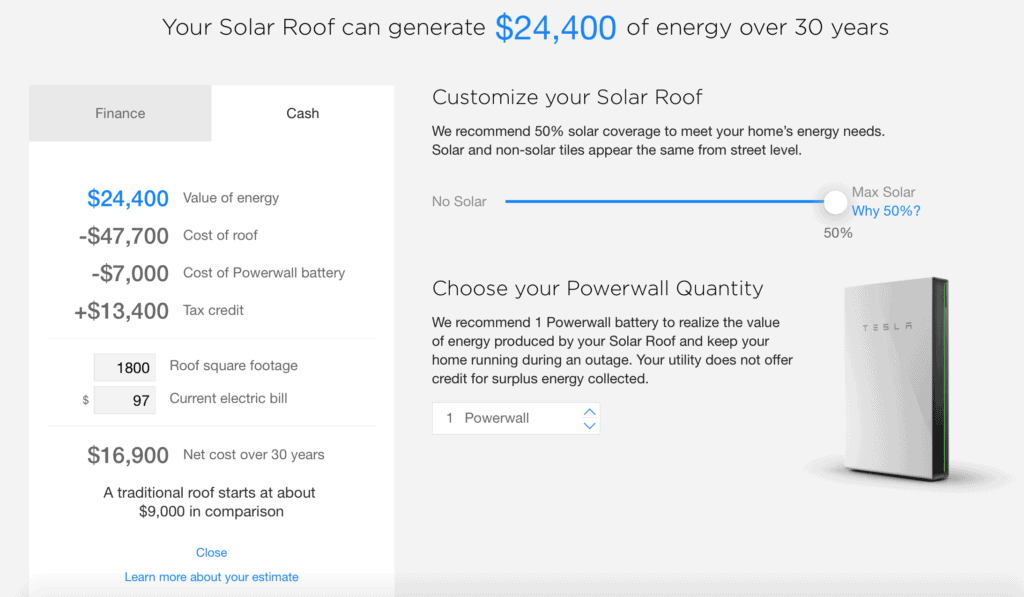The image features a light gray background at the top with text layered over it. Starting from an inch from the left, black lettering reads "Your Solar Roof Can Generate," followed by a blue "$24,400" and concluding with "in energy over 30 years" in black. On the left side, there's a white rectangle with two tabs at the top: a gray tab labeled "Finance" in black text, and a white tab labeled "Cash" also in black text. 

Below this, on the left side, there are monetary figures listed downwards. The first figure is in blue, with the following three in black. These lines show the footage, current electric bill, and net cost over 30 years. To the right of these figures, there's a breakdown of the value of energy, cost of the roof, and additional pricing details.

Below these details, text in black states, "A traditional roof starts at about $9,000 in comparison," with "Close" in blue beneath it. Further below, another blue text says, "Learn More About Your Estimate."

To the right, next to the word "Generate," starting at the "R," black text reads "Customize Your Solar Roof." Below this, there are two lines of information followed by the text "No Solar." A blue line extends from this point to about two inches from the right, ending in a white circle. Underneath the white circle, it says "50%," and to its right, "Max Solar" is written in black, with "Why 50%?" in blue below it.

Near the bottom of the image, there is a square with the Tesla logo on the front and a black spine on the right side. To the left of this square, large text reads "Choose Your Powerwall Quantity," followed by four lines of description. Lastly, there are two rectangles; the larger one is white, containing a smaller black rectangle inside it with "Powerwall" written in black.